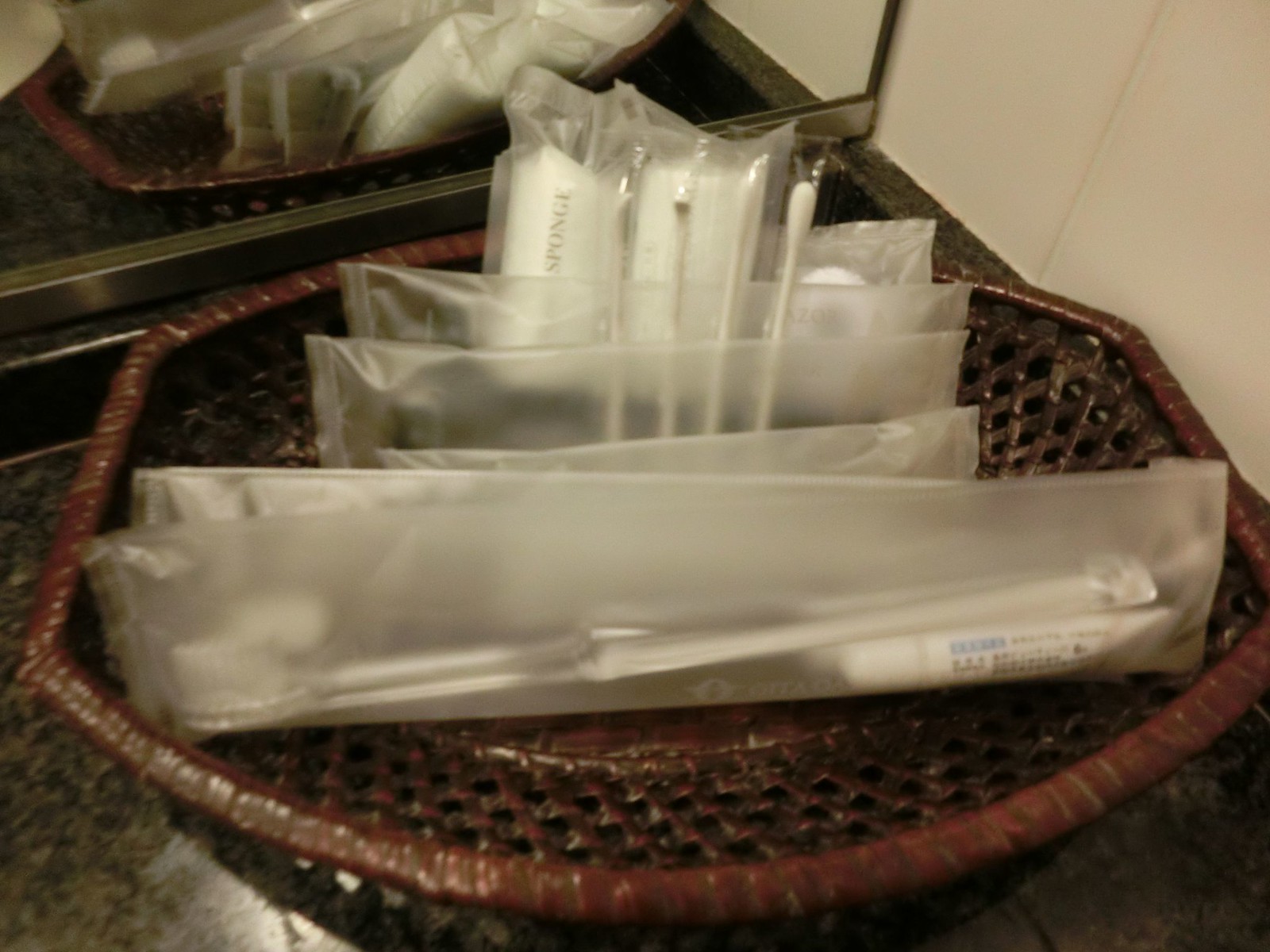This photograph appears to be taken in a bathroom, featuring a standard, thin-framed mirror on the back edge of a dark gray, marble-textured countertop. On the counter lies a sturdy, dark brown wicker basket. The basket contains several translucent white plastic baggies, each individually wrapped with various toiletries. Visible items in these baggies include a clear toothbrush paired with a small tube of toothpaste, individually wrapped Q-tips, a bar of soap, cotton pads, and possibly even a wrapped mint. The bags are small and arranged in a way that prevents a clear view of every item, but the presence of hygiene essentials suggests this setup could be for guest use, reminiscent of accommodations provided in hotels.